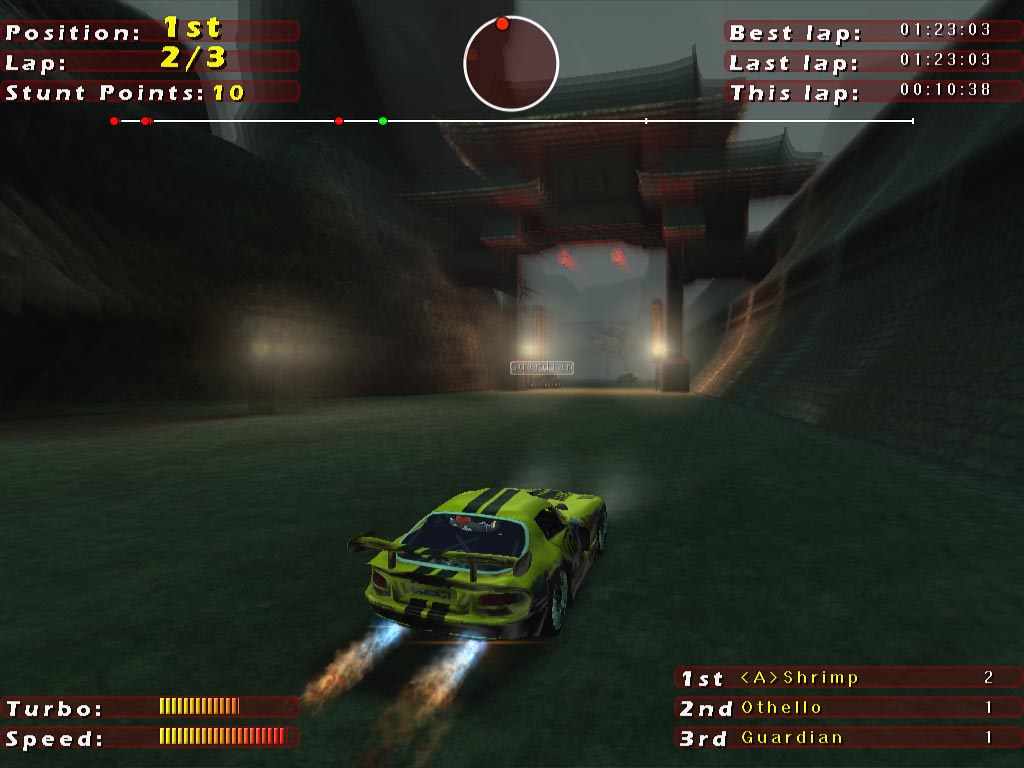In this vibrant screenshot of a racing video game, possibly from the Need for Speed franchise or a similar title, the action unfolds in a visually striking setting reminiscent of an Asian temple, potentially in Japan. The primary focus is on a dynamic yellow sports car adorned with two black stripes running down its center and a prominent rear wing. Blue flames burst from its exhaust pipes, suggesting high-speed motion.

In the HUD (Heads-Up Display), positioned in the upper left corner, three red, semi-transparent stripes provide crucial race information: "Position: 1st" in white and yellow, "Lap: 2 of 3" in white and yellow, and "Stunt Points: 10" also in white and yellow. Opposite this, in the upper right corner, three more red stripes display lap times: "Best Lap: 01:23.03," "Last Lap: 01:23.03," and "This Lap: 01:00.38" all in white text. Additionally, a round minimap centered on the screen shows various racer positions with red and green dots marking their locations.

The foreground details a concrete-like race track with green hues, bordered by intricately designed walls reflecting Asian architecture, complete with characteristic multi-layered, curved roofs. A white line runs almost the entire length of the image under the HUD, adding to the layout's clarity. At the bottom left, a turbo meter appears three-fourths filled, transitioning from yellow to red, indicating the car's boosted speed. On the right, a standings list displays racers with names in yellow and their respective positions in white.

The image impeccably captures the thrills of high-speed racing in a visually captivating, thematically rich environment.